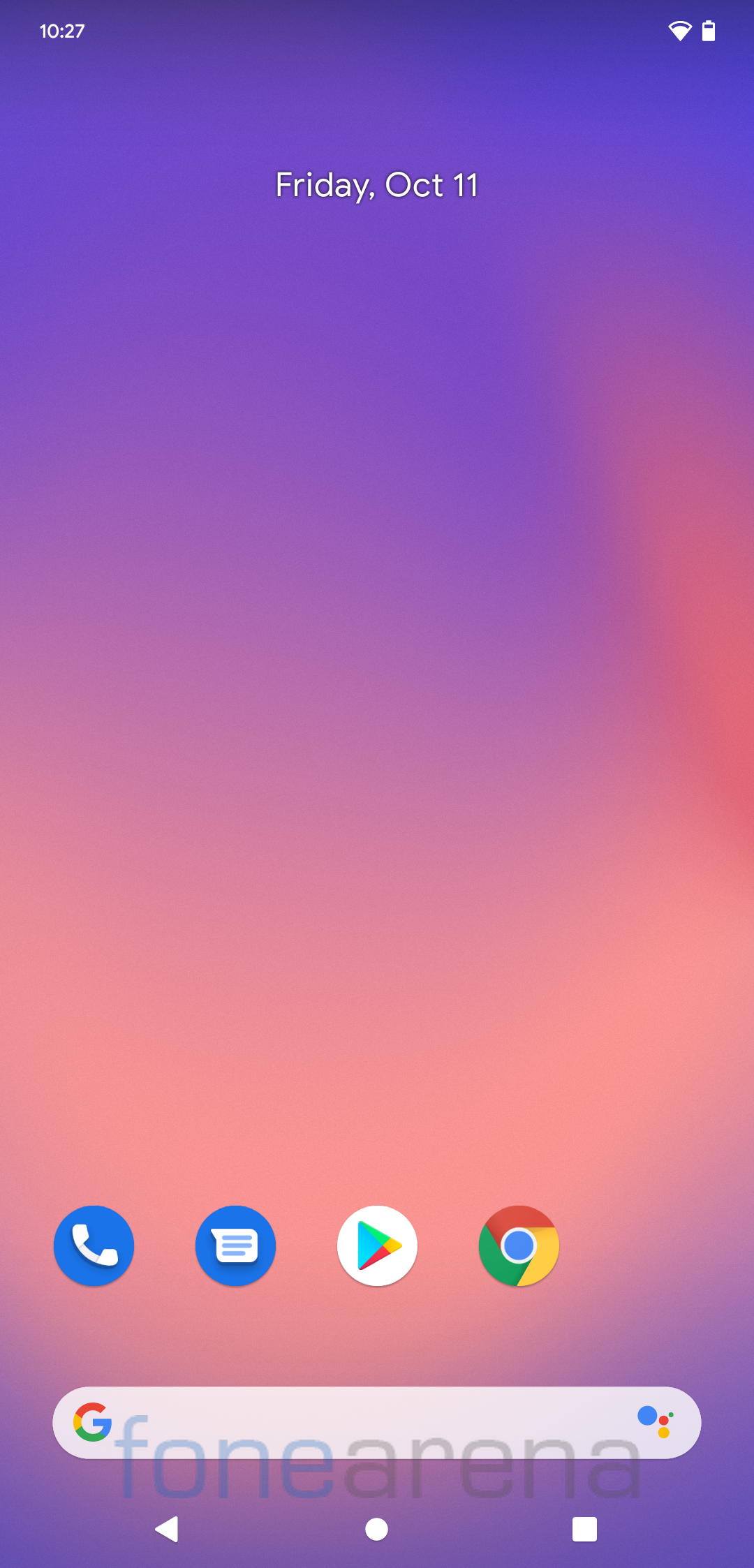This image showcases a smartphone home screen with a vibrant and eye-catching wallpaper. The wallpaper features a gradient blend, starting with a deep purple at the top that transitions smoothly into a pinkish hue, and then into a vivid orange in the center. Towards the bottom, the gradient transitions back into a rich purple. 

At the bottom of the screen, there's a navigation bar with three white icons: a back arrow, a circle for the home button, and a square for recent apps. 

A gray search bar adorned with the colorful Google logo and the Google Assistant logo sits near the top of the screen. Below the search bar, several app icons are visible, including Messaging, Google Play Store, Google Chrome, and the Phone app.

A watermark from Phone Arena, with "FONE" in blue and "ARENA" in gray, is also visible. The status bar at the very top displays the time as 10:27, alongside icons for Wi-Fi and battery life, and the date, "Friday, October 11th."